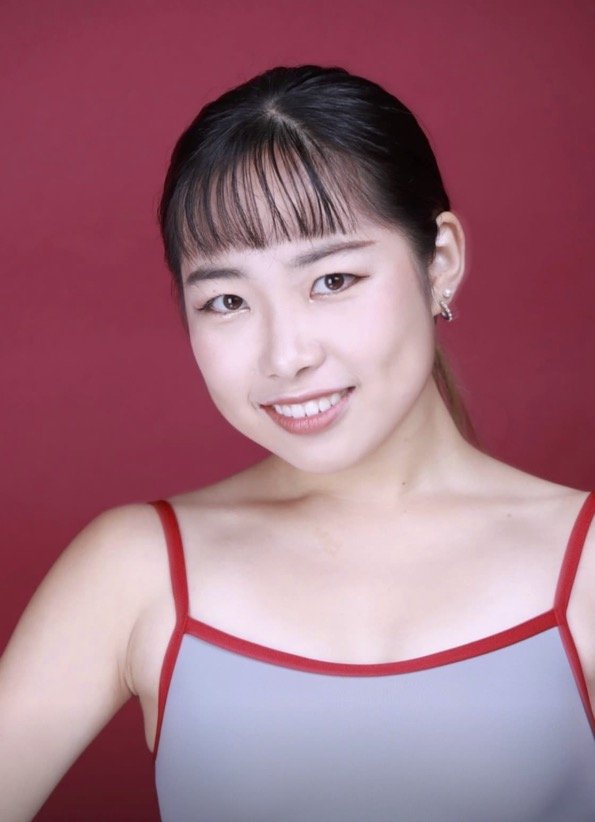The image showcases a young Asian woman with light-colored skin, depicted from the chest up against a solid red background. She has long black hair styled with bangs and is smiling, revealing white teeth. Her dark brown eyes are framed by minimal, natural-looking makeup, emphasizing her natural beauty. She wears two distinct earrings: a small pearl stud and a slightly larger hoop earring. Her attire consists of a gray tank top with thin red spaghetti straps and red edging. The lighting seems to be well-balanced, possibly illuminated from behind the camera, making her the focal point of the image. She appears content and is likely in her early twenties, exuding a poised and photogenic presence akin to glamour or acting headshots.